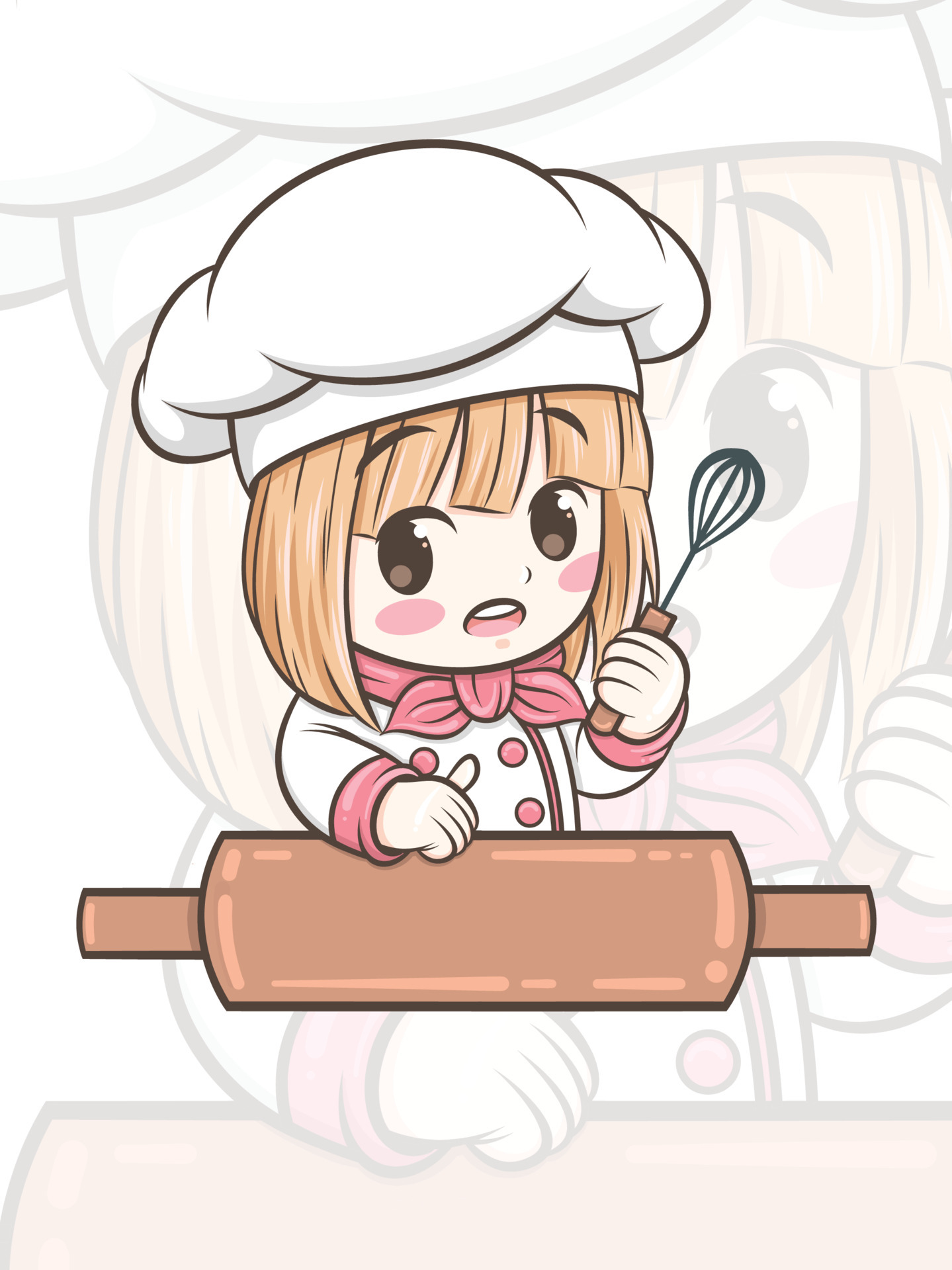This image, rendered in a Japanese manga-inspired kawaii anime style, depicts a young girl dressed as a chef. She has short, straight blonde hair with bangs, and her expressive features include large eyes and a small, slightly open mouth with pink lipstick and a hint of blush on her cheeks. She wears a classic white chef's hat and a white chef's jacket adorned with pink cuffs, three pink buttons, and a pink bow tied securely around her neck. With one hand, she holds a whisk, and the other rests on a large brown rolling pin. The overall colors are simple and few, emphasizing her light blonde hair, white attire with pink accents, and the brown rolling pin. In the background, there is a larger, transparent version of the same image, suggesting versatility in sizing and coloring for the clip art. This stylized depiction captures the essence of cute and youthful charm, characteristic of anime art.